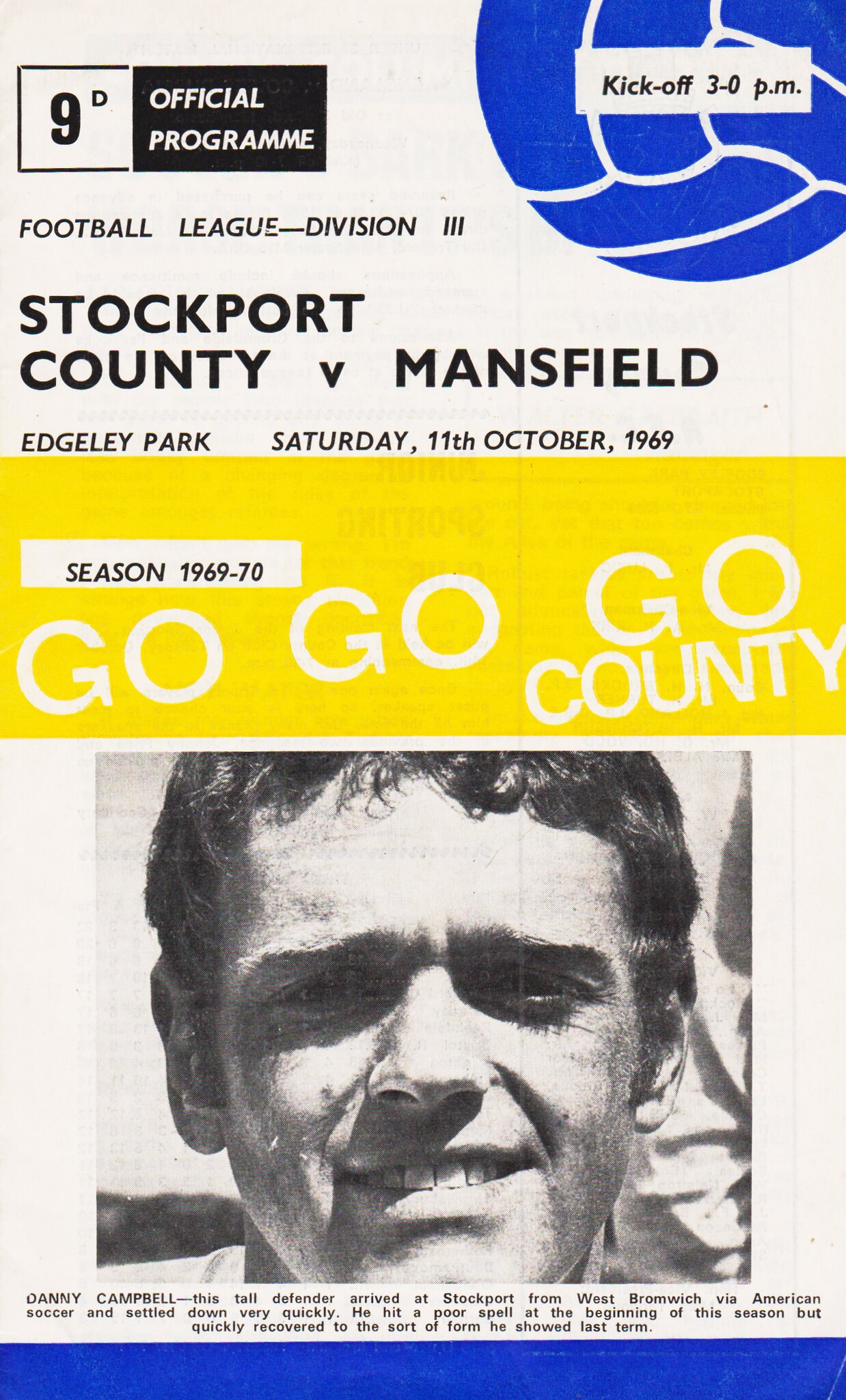This vintage soccer program cover from the 1969-70 season features a detailed monochromatic design with vivid spot colors in blue and yellow. The background is light gray. In the top right corner, a blue-outlined soccer ball with a white banner reads "kickoff 3-0 pm" in lowercase black text. At the top left, a black banner with white text proclaims "official program," accompanied by a white box labeled "9-D." Beneath these elements, the text "Football League Division 3" appears in bold black capital letters, followed by "Stockport County v Mansfield." Below this, in smaller black print, the location "Edgley Park" is specified along with the date "Saturday, 11th October, 1969."

In the middle section, a wide yellow banner features the enthusiastic exhortation "Go Go Go County" in white diagonal text, alongside a white inset declaring "season 1969-70" in black. The lower half of the cover displays a black-and-white photograph of a man facing the viewer, identified as Danny Campbell, with a paragraph of text describing him. A blue horizontal band runs across the bottom, adding depth to the classic design of this nostalgic football program.